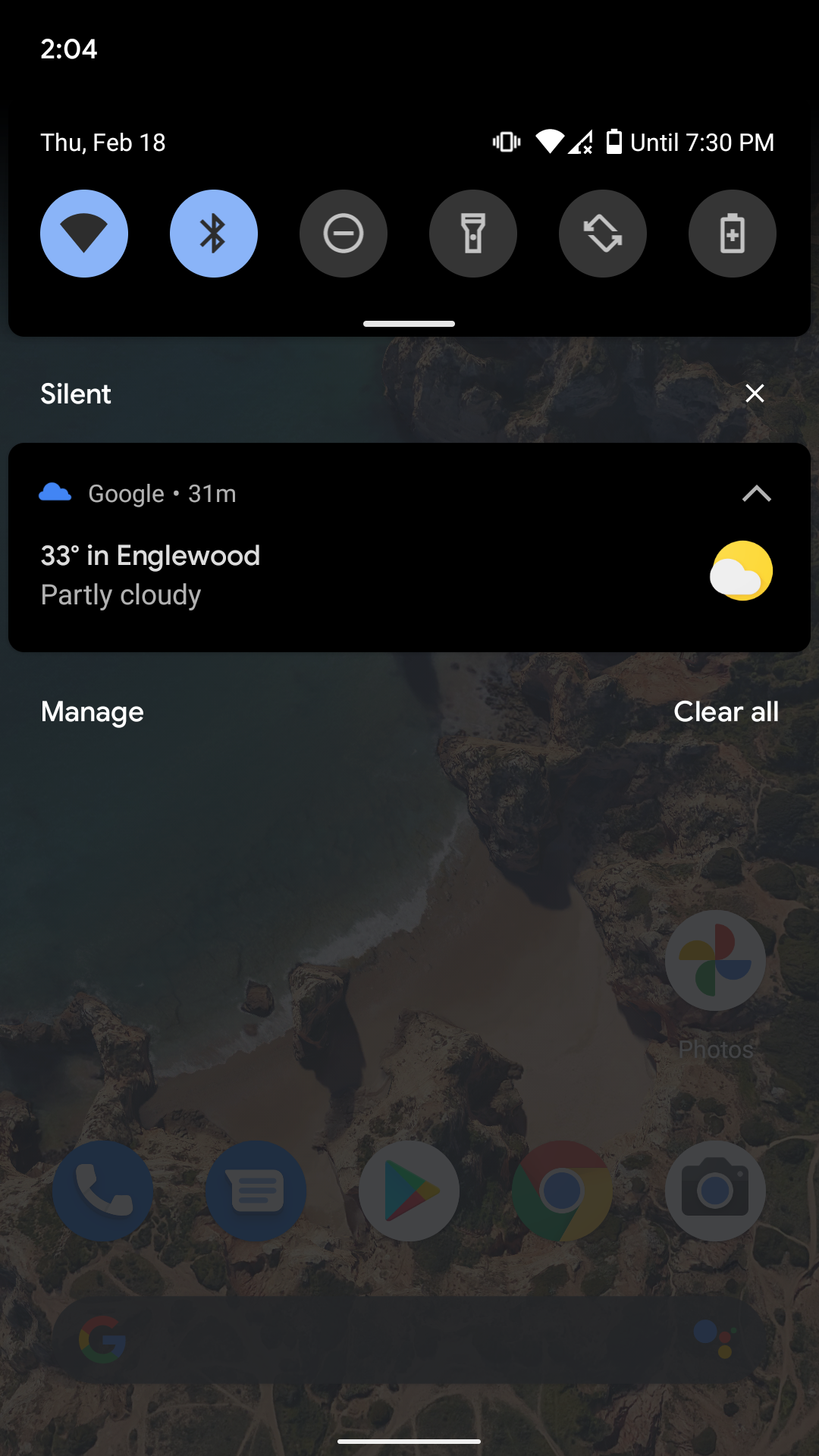This image captures a phone screen displaying several layers of information. At the top of the screen, the time is shown as 2:04 PM on Thursday, February 18th. To the left, various status icons are visible, including a shaking phone icon, a Wi-Fi icon, a network signal icon, and a battery icon indicating power until 7:30 PM.

Directly below these icons, a set of control buttons are displayed, including toggles for Wi-Fi, Bluetooth, Do Not Disturb, and Flashlight, along with a battery status button. Further down, the screen indicates the phone is in silent mode.

Just below these control buttons, a notification from Google provides the current weather update, showing a temperature of 33 degrees Fahrenheit and indicating that it is partly cloudy.